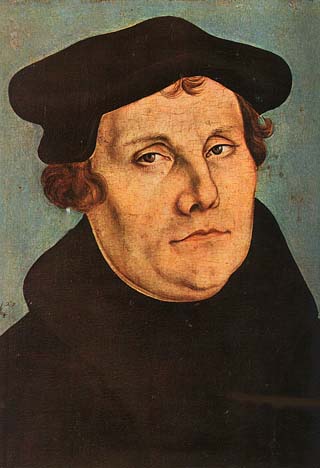This is a color painting of Martin Luther, likely from the early 1500s. Martin Luther, a white man, is depicted in a forward-facing pose, wearing a small, black cap. His hair is reddish-brown and slightly curled, visible from both sides of his head and the top. He has a prominent nose and a double chin. His dark clothing, reminiscent of a cowl-neck shirt or sweater, covers him up to the neck. Luther's eyes are directed to the left, and his mouth is closed, revealing a small dimple in his chin. He has a full face with some shading on his cheeks, indicating a larger build. The background is a muted gray color, providing contrast and focus on his detailed features.